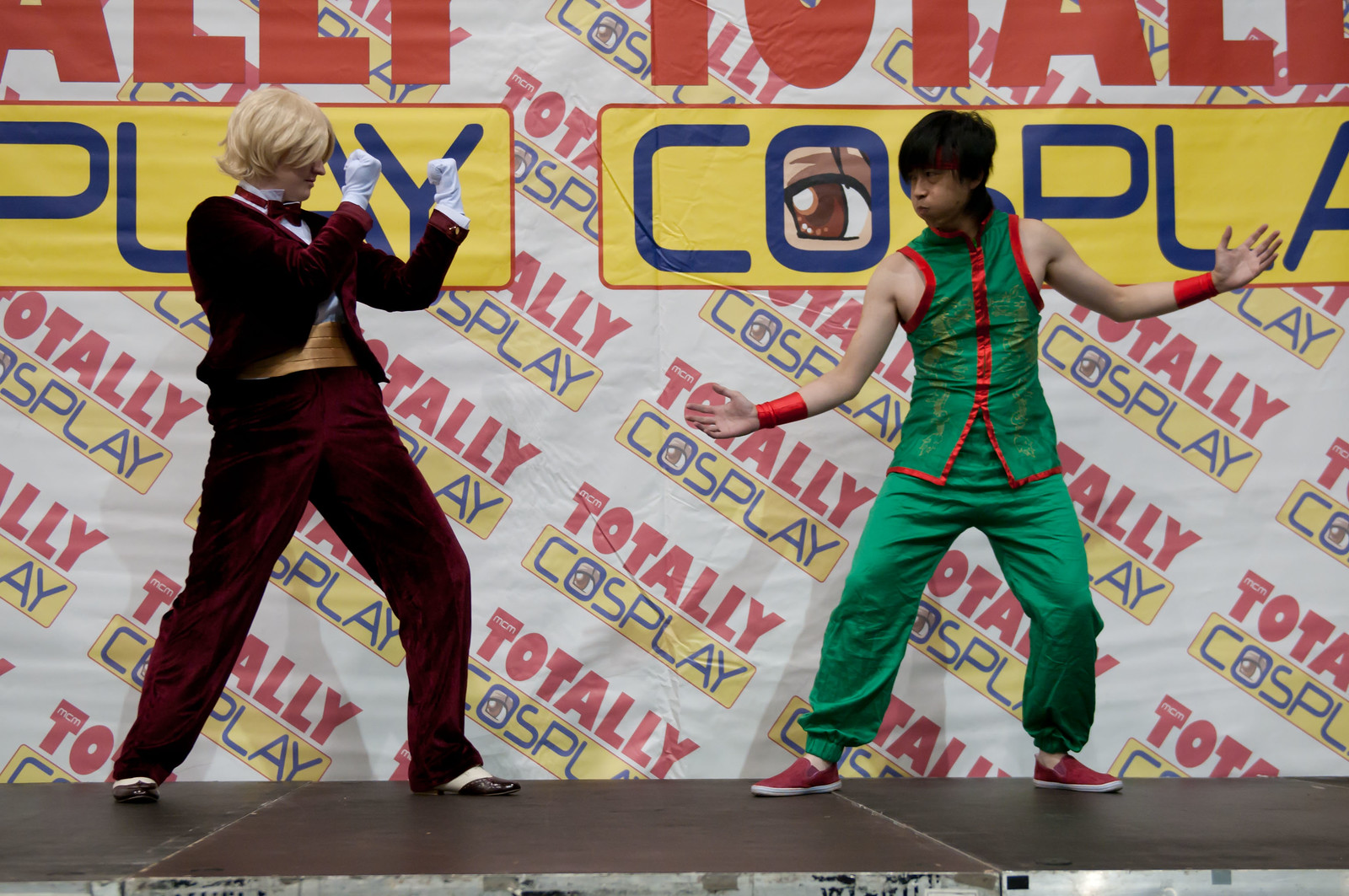In this photograph, two individuals are striking a playful pose in front of a backdrop emblazoned with the words "Totally Cosplay." The backdrop features "totally" in red lettering, and "cosplay" with a yellow background and blue lettering. The scene appears to be set on a platform, giving the image a staged feel.

The person in the foreground appears to be a woman. She sports a blonde wig, a velvet burgundy outfit adorned with a gold band around the waist and a matching dark velvet bow tie. She completes the look with white gloves and black-and-white dress shoes. Her stance is defensive, with fists raised in a classic boxing posture.

To her right stands an Asian man, dressed in a green and red satin martial arts-inspired costume. His attire is accented with red wristbands and matching red shoes. He adopts a dynamic pose, legs and arms spread wide, with his face and cheeks puffed up as if ready to engage in a mock fight.

The overall composition captures the essence of cosplay, with both participants fully immersed in their character roles, making it a lively and engaging scene.